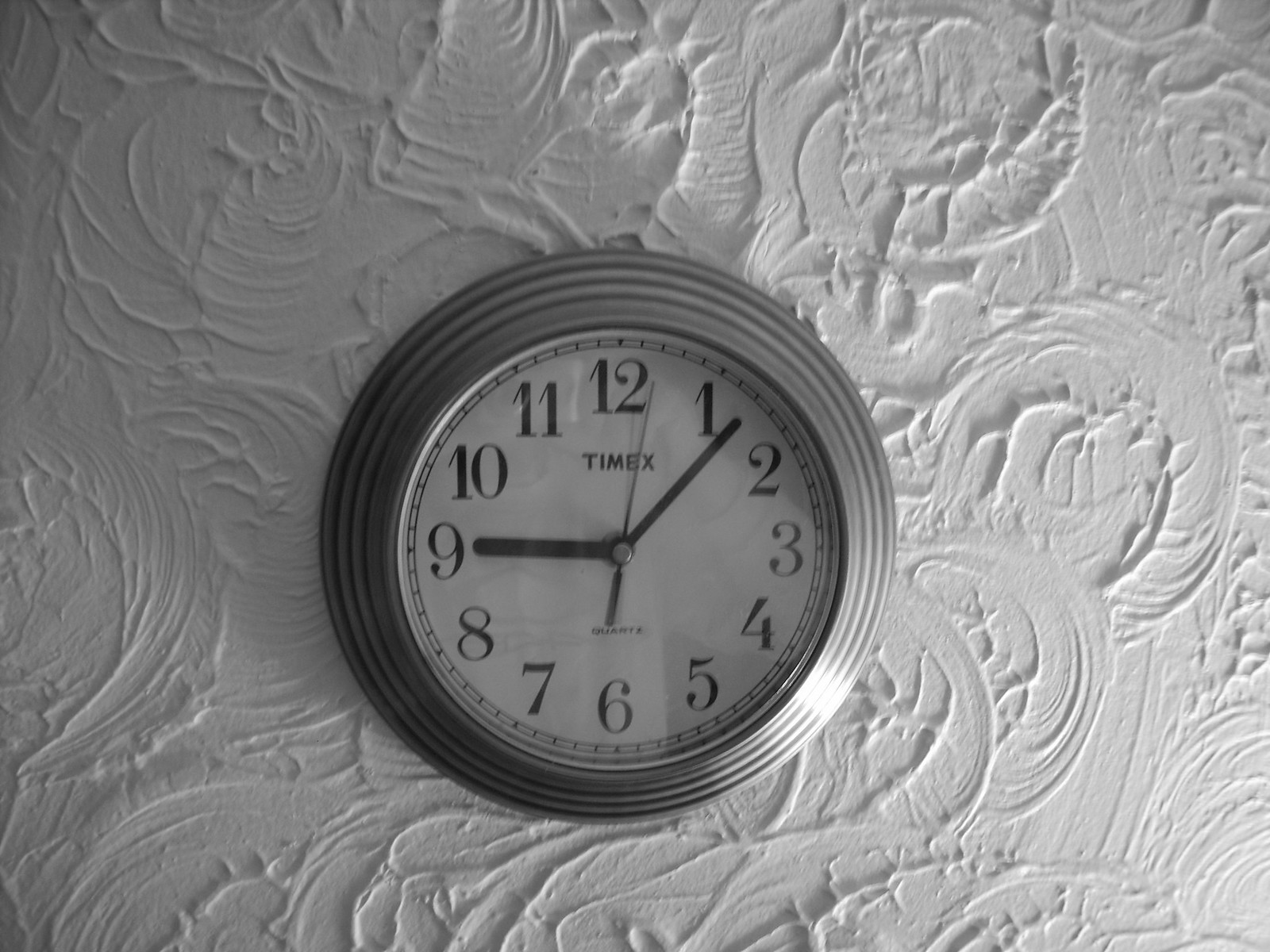The color photograph features a Timex wall clock mounted on a distinctively textured white wall. The wall is covered in swirling patterns and veiny circular designs that give it a highly tactile appearance. The lighting casts a shadow on the upper left portion, with more illumination coming from the bottom right, enhancing the wall's texture. The clock has a thick, tiered gray frame that almost makes it appear silver. Its face is white, with bold black Arabic numerals from 1 to 12, and the word "TIMEX" prominently displayed in black just below the 12. Black minute and hour hands, along with a black second hand slightly past the two-second mark, show the time as 9:07. Despite its purpose, the clock blends in somewhat with the similarly colored wall, rendering the overall scene rather plain and uninspiring.